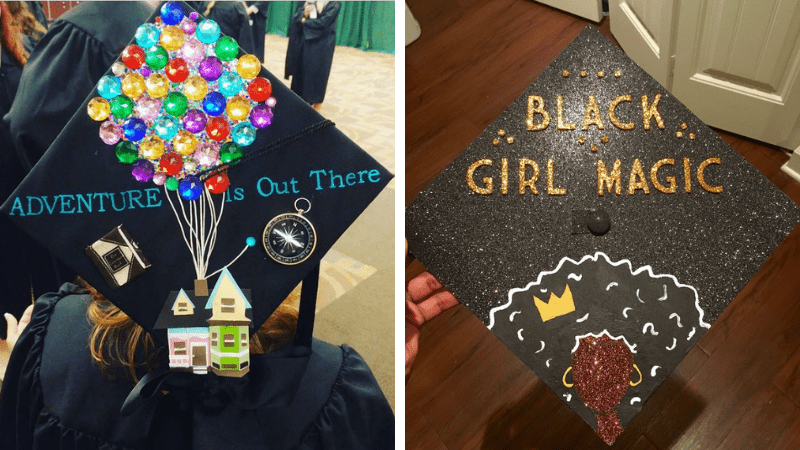The left image showcases a graduation cap decorated with a captivating theme from the movie "Up." Viewed from above, the cap features a house with brightly colored balloons—red, green, blue, yellow, and purple—floating upward from its chimney. The balloons are intricately crafted from pom-poms and string, enhancing the cap's texture. Supplementary details include a compass and a camera, intricately placed alongside the text “Adventure is out there,” alluding to a sense of exploration and journey.

The right image displays another creatively adorned graduation cap, positioned in a diamond shape. The cap exudes elegance with its glittery backdrop and raised gold-lettering proclaiming, “Black Girl Magic.” Set against a wooden floor in a home interior with white walls, the cap also features a striking illustration of a black woman, her large hair, golden earrings, and a gold crown epitomizing regal beauty and empowerment. The combination of the cap's dazzling glitter and powerful message captures the essence of pride and celebration.